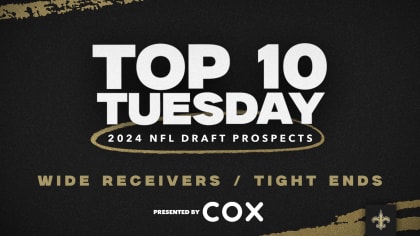The image features a predominantly black rectangular football banner with intricate detailing. Across the middle, bold white text prominently reads "Top 10 Tuesday," exuding confidence and emphasis. Directly beneath this, in a smaller white font, are the words "2024 NFL Draft Prospects," encircled by a hand-drawn, oval-shaped outline in a bronze-tan hue. Below, in the same bronze-tan color, bold and slightly larger text states "Wide Receivers / Tight Ends." At the very bottom, in small white font, "Presented By" appears, followed by "Cox" in significantly larger, bold white letters and a smooth, Sans Serif style. The banner also has distinct khaki-colored grungy line accents in the upper left and bottom right corners, adding a unique design aspect. Additionally, off to the right side, there is a decorative emblem that resembles a stylized fence with a pointed top and branch-like wings descending, anchored by a base.